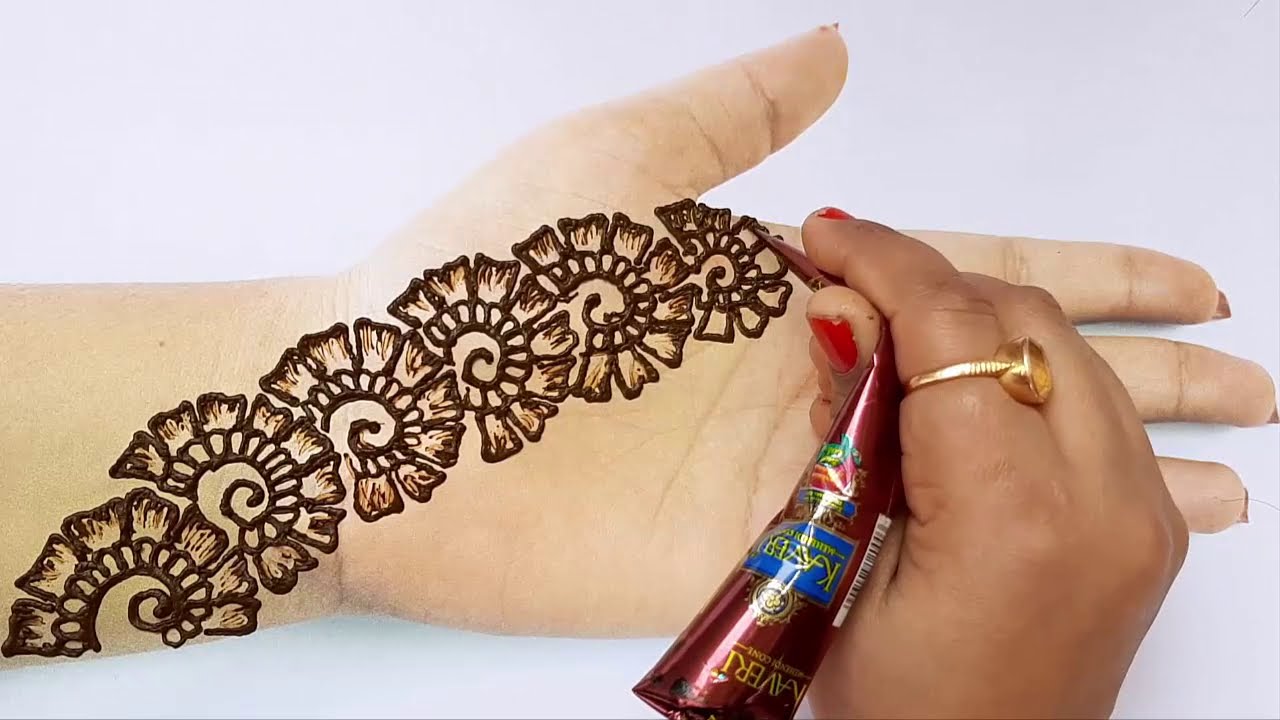The image depicts a woman intricately designing a henna tattoo on her left hand, which is positioned palm-up on a white surface. Using her right hand, she squeezes dark brown ink from a plastic tube with a pointed tip. The tube has a red and blue logo on its plastic cover. The woman's fingernails are painted red, and she is wearing a gold ring on her right index finger. The henna design features a repetitive, flowery pattern with six flowers, each having seven petals and intricate swirls in the middle, extending diagonally from the wrist up to just below the thumb. The detailed artwork combines half-circles, spirals, and ovals to create an elaborate, flower-like motif that runs across the wrist and forearm.